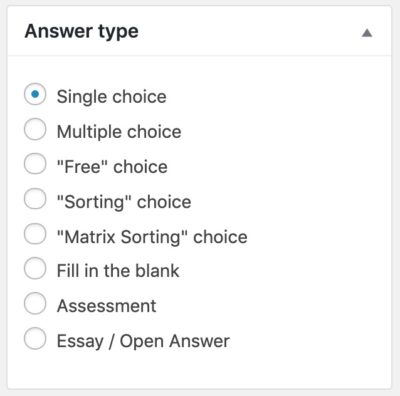The image depicts a form with a heading labeled "Answer Type" in bold text, accompanied by an upward-facing gray arrow. The form has a white background, framed by a thin gray border, and it bears a rectangular shape. Below the heading, there is a vertical list of eight selectable options, each represented by a white circle that can be filled with a blue dot when selected.

Currently, the first option "Single Choice" is selected, indicated by a blue dot inside the white circle. The subsequent options listed are:
1. Multiple Choice
2. "Free" Choice
3. "Sorting" Choice
4. Matrix Sorting Choice
5. Fill in the Blank
6. Assessment
7. Essay/Open Answer

All other circles are blank, signifying that they have not been selected.